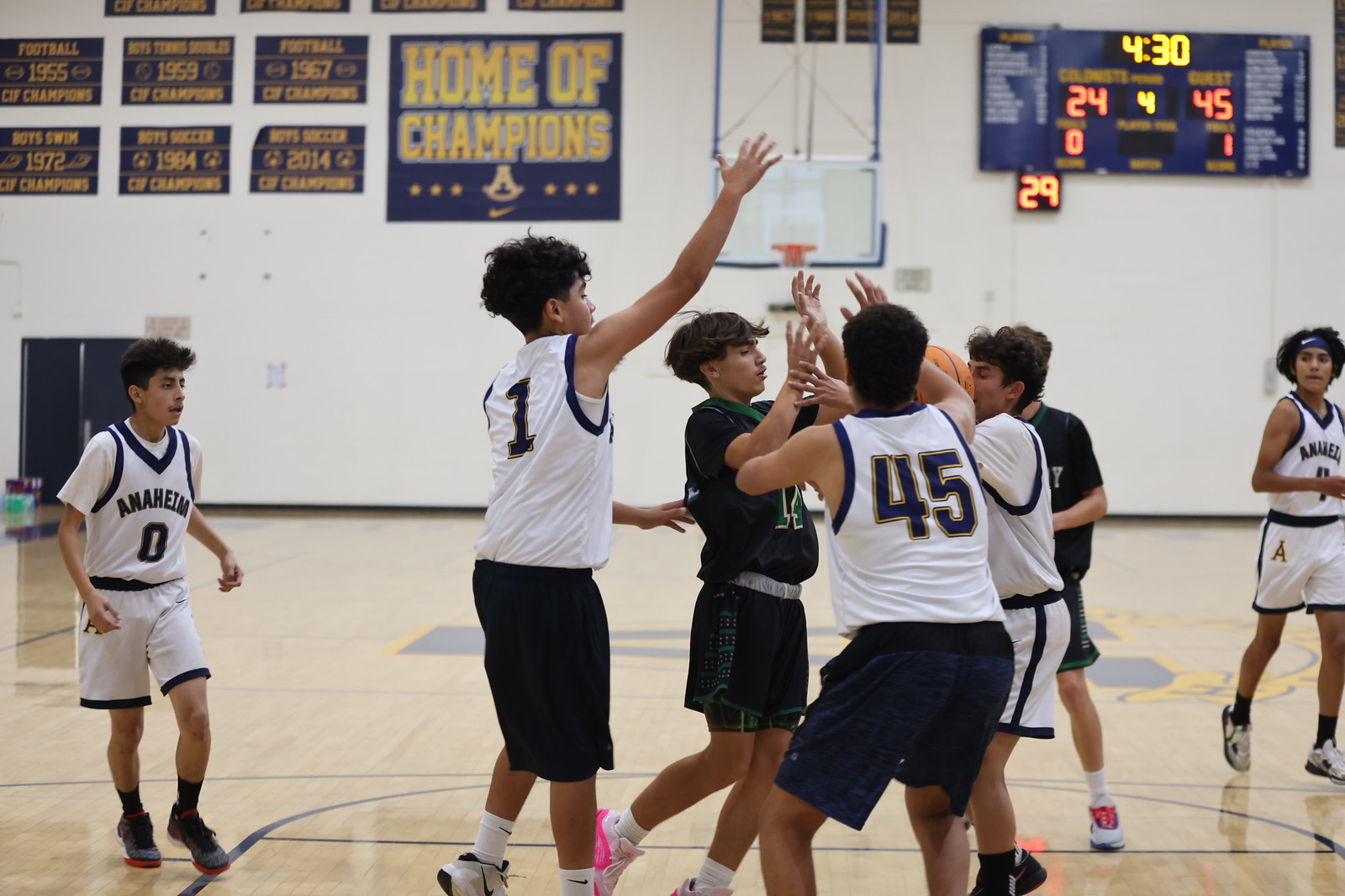The photograph captures a vivid scene of a high school basketball game in progress, featuring a group of young teenage boys intensely engaged on the court. Set in a well-lit gymnasium, seven players are seen clustered together on one side of the court, vying for control of the basketball. The teams are distinguishable by their uniforms, with one team donning white jerseys with navy blue letters and the other sporting black jerseys. In the background, the scoreboard indicates a score of 24 to 45, with four minutes and 30 seconds remaining in the game. Adorning the gym walls, several banners highlight the school's championship history, with years such as 1955, 1959, 1967, 1972, 1984, and 2014 prominently displayed. The gym's atmosphere is vividly captured, showcasing both the competitive spirit and rich history of the venue.